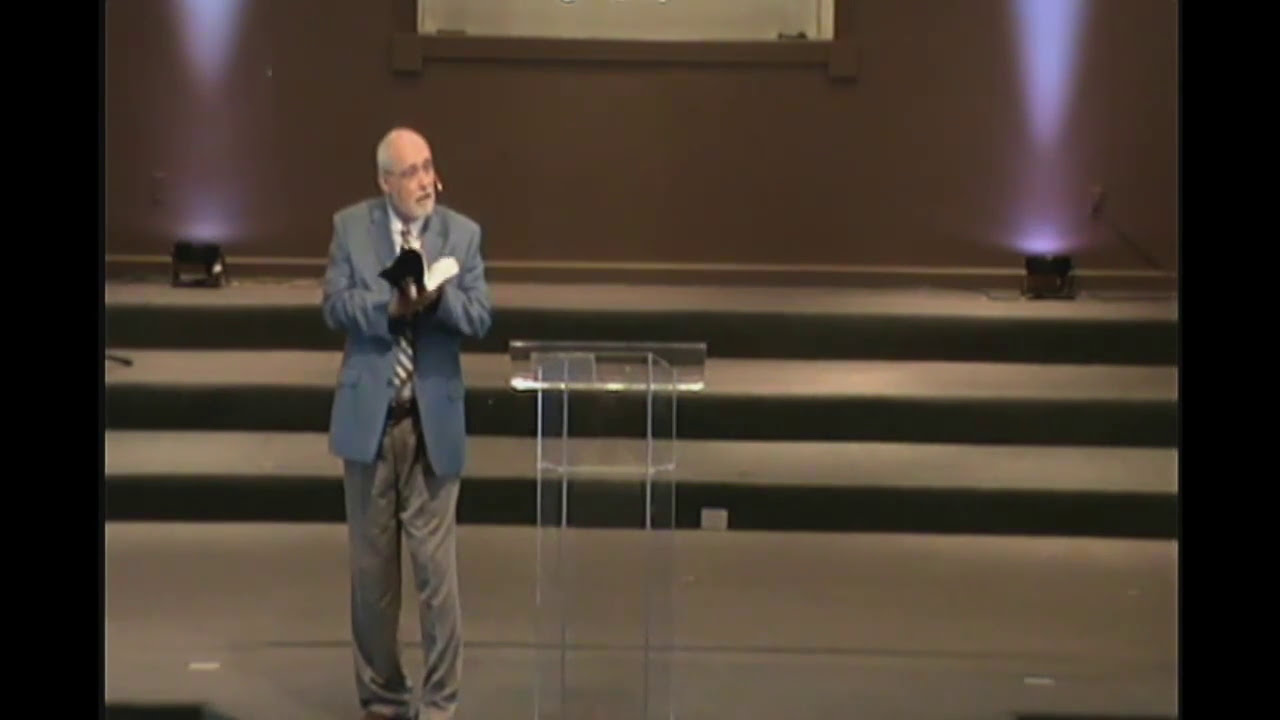In this indoor stage setting, an older man in his fifties stands towards the left side of the horizontally oriented photograph, seemingly mid-speech to an unseen audience. He faces the camera with a small microphone looped around his left ear, its boom positioned near his mouth. The man, balding with a ring of gray hair at his temples and a matching gray mustache and beard, is dressed in a gray suit jacket over a white shirt, complemented by a striped tie and tan trousers. His arms are bent at the elbows and crossed at his chest, holding a book. To the center-right of the image, just behind his left elbow, is a translucent glass podium supported by four thin legs. The stage features a purple backdrop accented by tower lights on either side, casting a whitish-purple glow upwards. Three wide steps, in shades of brown and tan, ascend from the wooden floor to the backdrop, creating a tiered platform behind him.